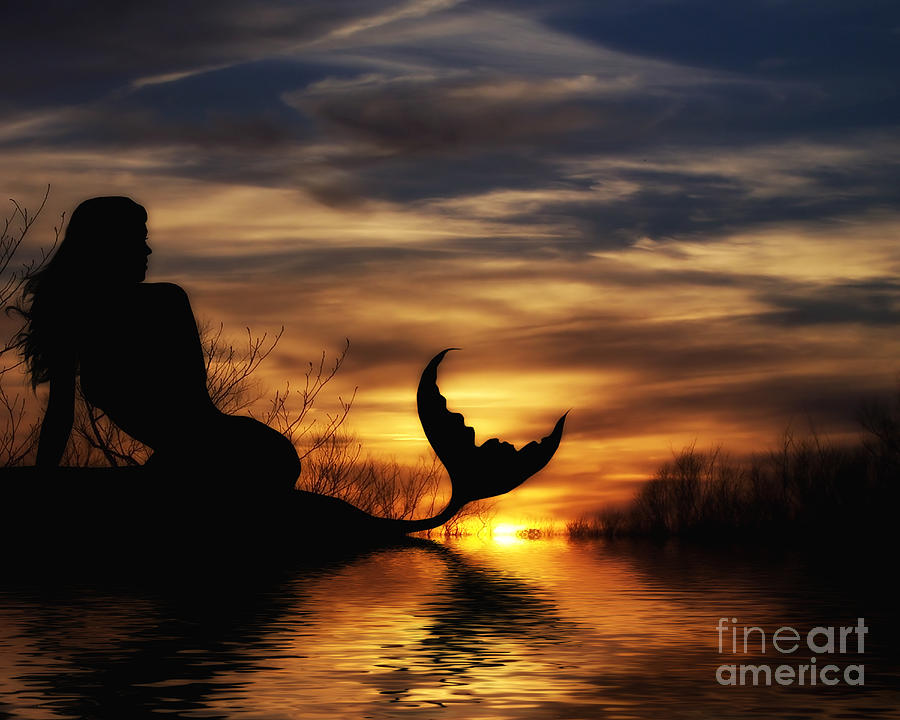The artwork, labeled "Fine Art America" in white text at the bottom right, depicts an enchanting outdoor setting at sunset. A central feature of the image is the silhouette of a mermaid with long hair and fine features, positioned on a small patch of grass near a golden-hued body of water in the left-hand side. The mermaid's tail is clearly visible, emphasizing her mystical presence. Surrounding the water are branches, bushes, and trees that frame the scene, adding depth and natural beauty. The sky above is a swirl of colors ranging from grey, dark grey, white, and hints of blue to light red, yellow, and brown, showcasing the dramatic transition of the sunset. The sun itself shines bright yellow in the background, casting a soft glow over the entire landscape and highlighting the serene yet mysterious atmosphere of this digitally created image.